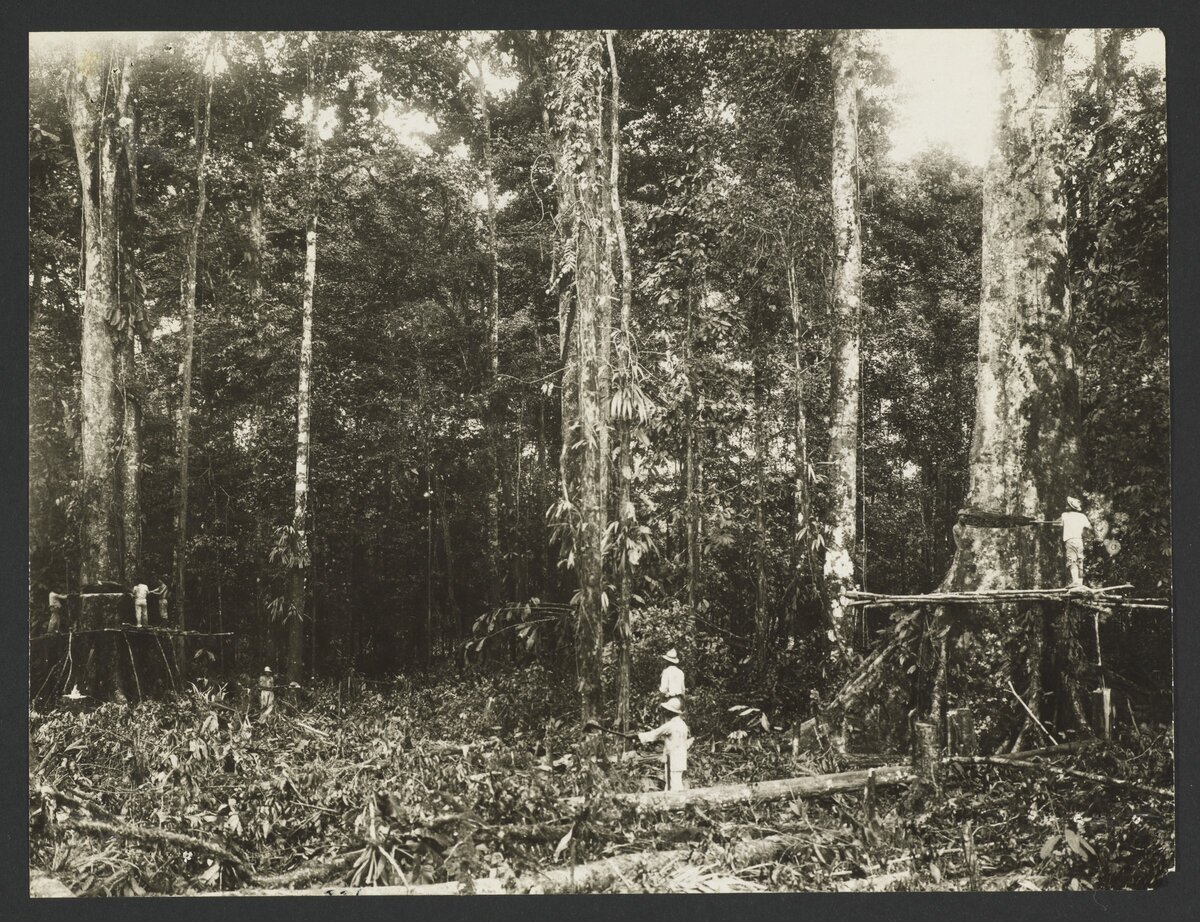This is a very old, black and white photograph, capturing the deforestation of an ancient forest, likely during the early 1900s or possibly the colonization period of India. The scene is densely wooded, possibly tropical, with gigantic trees being cut down for lumber. The photo is mounted on black cardboard and has a light sepia tone, giving it a brownish hue. 

At the forefront, three men, dressed in white outfits and domed safari-style hats, are using a large handsaw to cut through one of the colossal tree trunks. On the left and right sides, scaffolding has been constructed around similarly large trees. Additional men are standing on these scaffolds, holding opposite ends of another large saw. Debris and fallen tree trunks litter the ground below. 

In the center, amidst the fallen trees and debris, another man is visible, seemingly swinging an axe. The background of the photo, bathed in soft sunlight that creates a slightly foggy and blurry effect, contains many more trees, although they appear smaller in comparison to the giants in the foreground. The image captures a stark and poignant moment of labor-intensive deforestation, emphasizing the scale of both the trees and the efforts to bring them down.